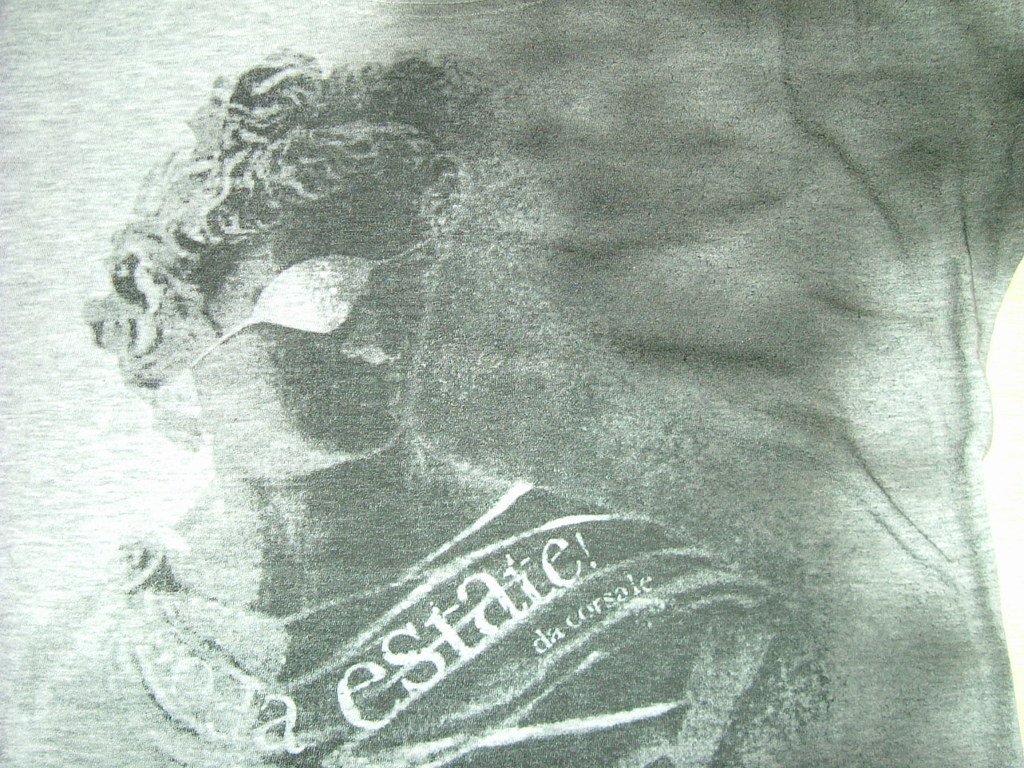The image, rendered in varying shades of gray, portrays a figure with short, tightly curled hair, and an eye patch. The individual stands facing the camera, but their head is slightly turned to the right, giving a sense of contemplative poise. Draped elegantly over their shoulder is a cloak, secured with a pin, adding a touch of regality to the composition. Emblazoned across the cloak in crisp white font are the words "Estate de Courcelles." Both the eye patch and the text stand out vividly in stark white, providing striking contrasts against the overall light gray and white palette of the image. The nuances of the grayscale tones lend a timeless and classic quality to the visual narrative.